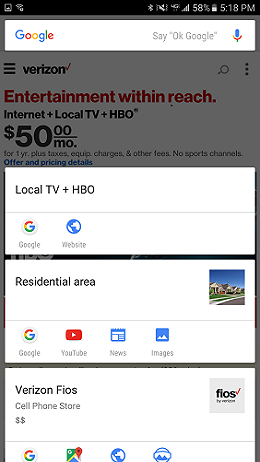A user is interacting with a Google app on their smartphone, with multiple interface elements visible. In the background, a dimmed browser window displays the Verizon website, advertising an entertainment package: Internet plus local TV and HBO for $50 a month, valid for one year with additional taxes. Overlaying this webpage, the Google app presents a search bar at the top, allowing voice commands via "Okay Google." The app appears to be contextually responding to the content on the Verizon site, likely providing supplementary information. At the bottom of the screen, there are several smaller app icons including Google Maps, along with links to news, images, YouTube, and other resources under different sections labeled "Fios" and "Residential area." The overall interface is somewhat cluttered and complex, making it challenging to discern the primary focus of the user's activity.